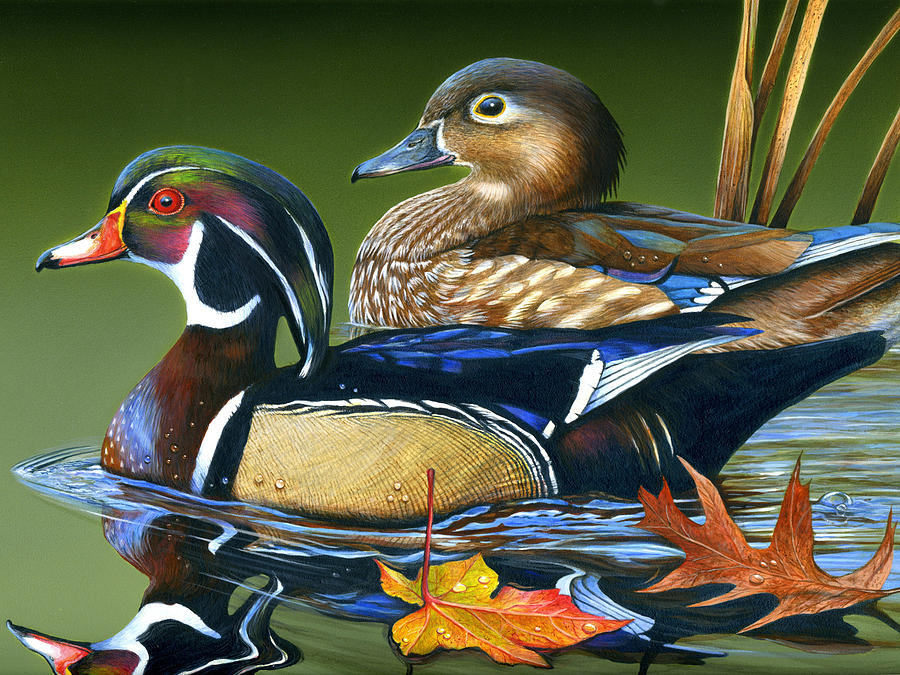This artwork depicts two ducks in a serene pond, exquisitely detailed and rendered with vibrant colors. The foreground features a larger, male duck distinguished by its striking green head adorned with a "mohawk" of green feathers, complemented by an orange bill and red eyes. His neck showcases contrasting black and white plumage, while his breast is adorned with rich maroon, brown, and blue shades. Golden and blue feathers accent his back, further enhancing his vivid appearance. His reflection is visible in the water, accentuating the clarity of the scene.

Beside him is a somewhat plainer but equally graceful female duck. She exhibits a predominantly brown and white feathering with subtle touches of blue on her back and near her tail. Her beak is gray, and she has a brown eye and a modest "mohawk" of feathers down her head.

The background transitions from a darker green at the top to a lighter green towards the middle and bottom, indicating a natural pond environment. Captivating reflections and ripples in the water evoke a sense of gentle movement, with two leaves and additional fall-colored foliage floating nearby. Completing the scene are hints of cattails and aquatic plants that enhance the natural beauty of this picturesque setting.